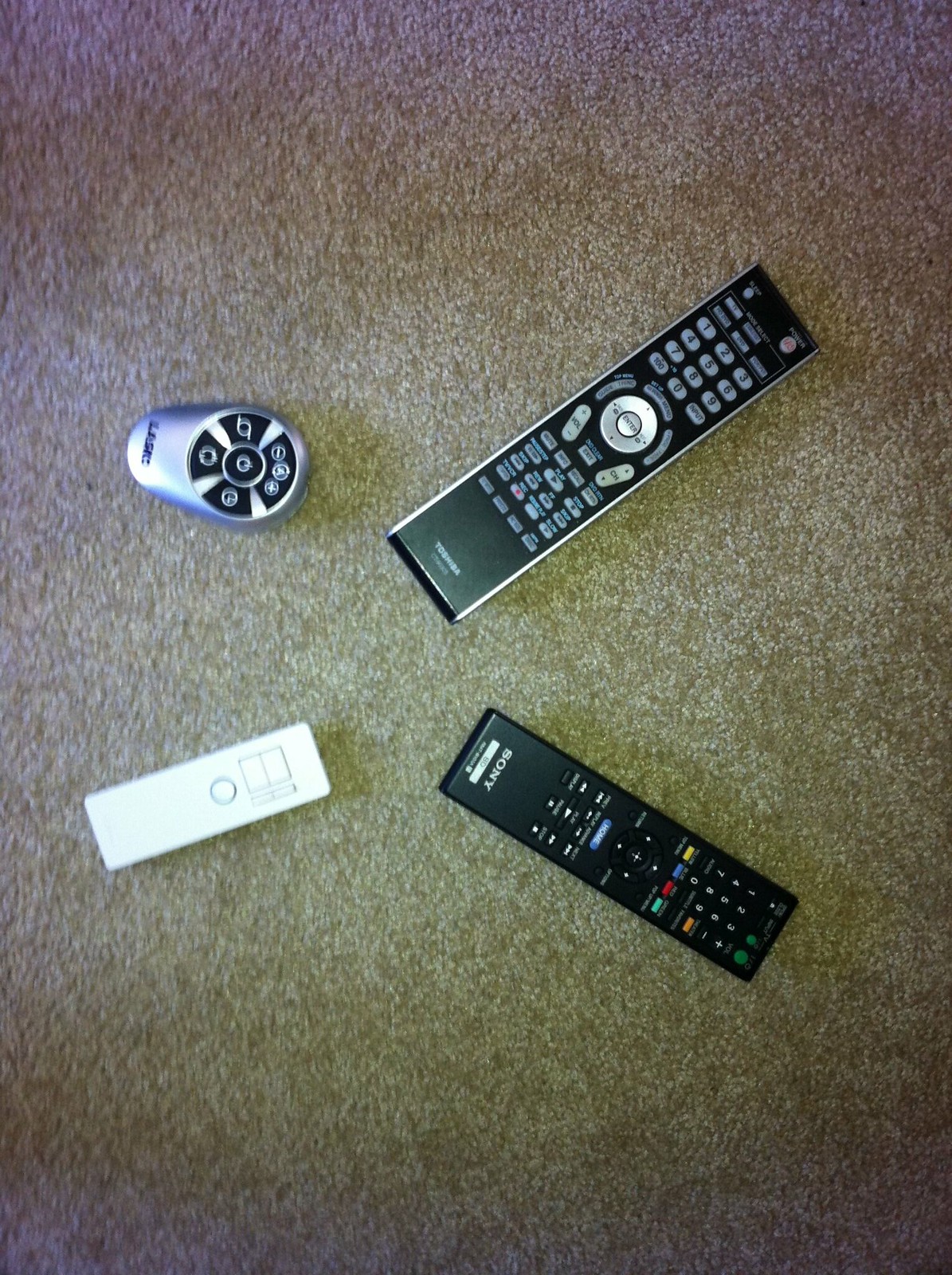The image showcases an overhead view of four distinct remote controls placed on a honey brown carpet. The lighting creates shadows at the top and bottom, with the center more brightly illuminated. On the upper left side lies a small, silver round remote, measuring approximately two inches in length, with a circular power button in the middle, surrounded by black and white buttons, and black text at the bottom. Below it, there is a slightly longer, white, rectangular remote with indistinguishable design details. To the right, there is a long, black rectangular remote, significantly larger than the others, branded "Toshiba" at the bottom, featuring a mix of gray and silver buttons, including circular control buttons in the center for volume and channel. Finally, angled down and to the right, is a black rectangular Sony remote with approximately 14-15 buttons, including a row of colorful buttons—yellow, blue, red, and blue—beneath black buttons marked with white numbers and letters.